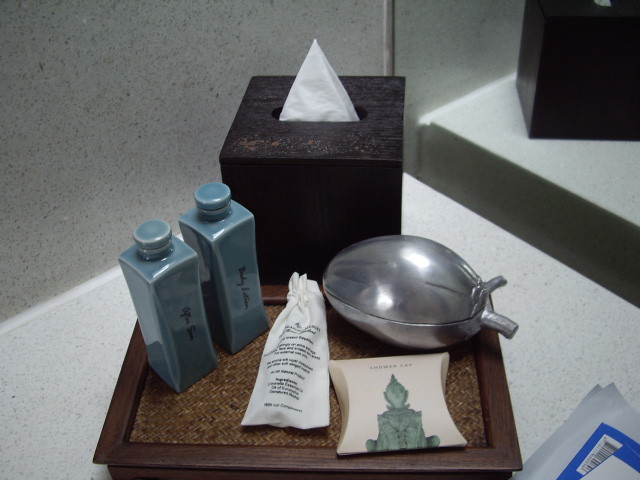The image captures a close-up of the corner of a hotel bathroom, showcasing a neatly arranged set of amenities. The background features a countertop and walls that are of a similar off-white color with specks of gray, giving a harmonious, speckled appearance. To the right, a mirror reflects a dark brown, wooden tissue box with a central slit and an elegant swirl design engraved on its front. A tissue, folded into a neat triangle, protrudes from the box, with the back of the box visible in the mirror.

In front of the tissue box sits a small wooden tray with a brown mat lining its base. This tray contains two blue bottles, possibly shampoo and conditioner, although the writing on them is not clearly legible. Next to these bottles is a small drawstring canvas bag with some writing on it, the exact contents of which are unclear.

Adjacent to the canvas bag is a silver object that resembles a bowl or perhaps a split-open mango. Its surface reflects light, and while its purpose is uncertain, the object adds a touch of intrigue to the arrangement. Below this, there is a distinctively shaped soap bar, square with inward-curved sides, featuring what seems to be an Asian temple or statue design engraved on it. Lastly, a small paper item is seen beside the soap bar, completing the array of toiletries and adding a final touch to this meticulously organized bathroom corner.